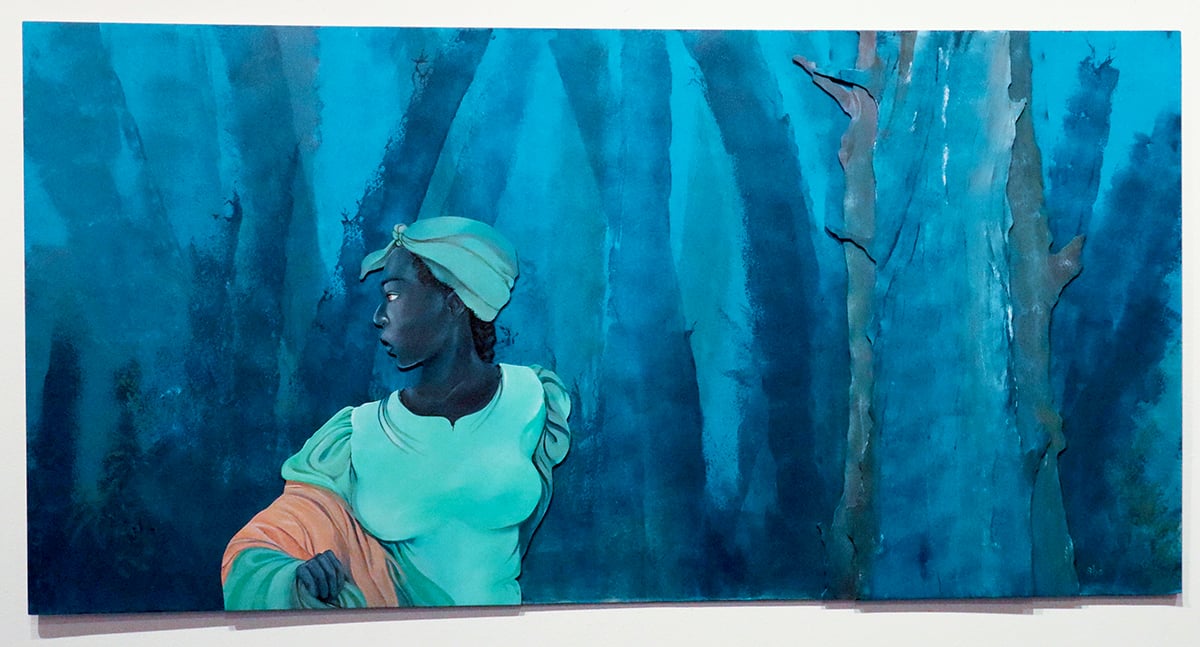This watercolor painting portrays an African-American woman in her twenties, captured in a moment of palpable anxiety. She is dressed in a teal head wrap and a teal dress, accented by a peach shawl draped over her right arm, which is extended and bent at the elbow. A hint of her black hair peeks out from under the head wrap. The woman’s body faces the viewer, but her head is turned to the right, her gaze filled with concern as if she fears being followed. The painting is set against a backdrop of dark blue and black tree trunks, devoid of leaves, creating an abstract, nighttime scene that heightens the sense of urgency and unease. The whites of her eyes are prominently visible, emphasizing her heightened alertness.